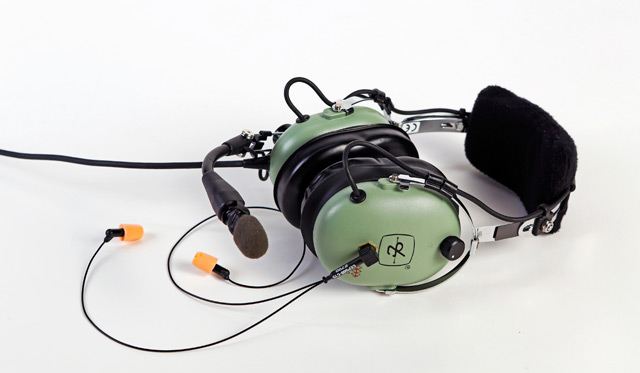This image depicts an aviation pilot's headset resting on a plain white surface with a white background. The headset is partially on its side, revealing several distinctive features. It is predominantly black and green, with large ear cups that cover the outer ear. The ear cups, sporting a mix of black and light green, have plush borders to ensure comfort. On the right ear cup, there is a black, curved microphone ending in a brown foam piece. A thick black wire is seen connected to the headset, extending from the left side. Additionally, there are two thin cords emerging from one of the ear cups, each terminating in small orange earplug-like points, suggesting an optional in-ear setup. The headband of the headset is black, featuring a sponge-like cushioning for added comfort. There's also a logo present on one of the ear cups, described as a square with a design in the middle. The overall layout of the headset, along with its detailed components, clearly indicates its specialized use for aviation purposes.